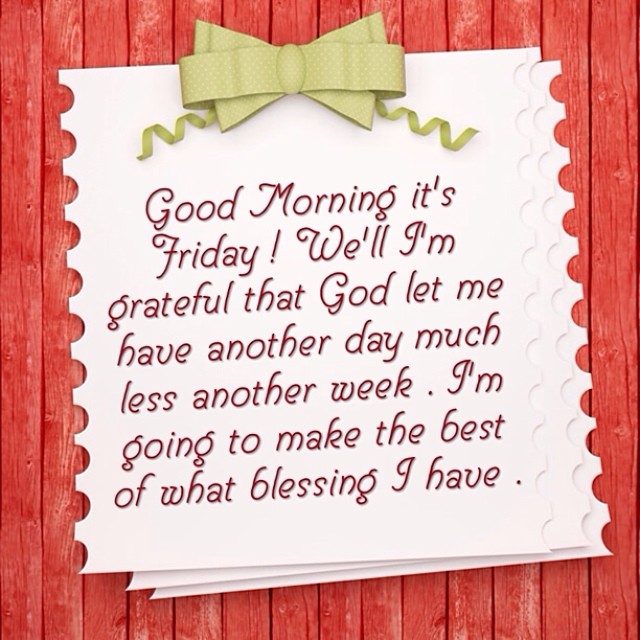The image showcases a thoughtfully designed graphic with a skeuomorphic touch, featuring a red-painted wooden plank background that resembles deck slats. At the center, a stack of three digital cards is layered, each with semicircular perforations along the sides. The top card displays a cheerful message in a playful semi-cursive font: "Good morning, it's Friday! I'm grateful that God let me have another day, much less a week. I'm going to make the best of what blessing I have." Completing the design, a light green and white polka dot bow tie adorned with spiraling streamers gracefully rests at the top of the stack, adding a whimsical touch to the overall composition.